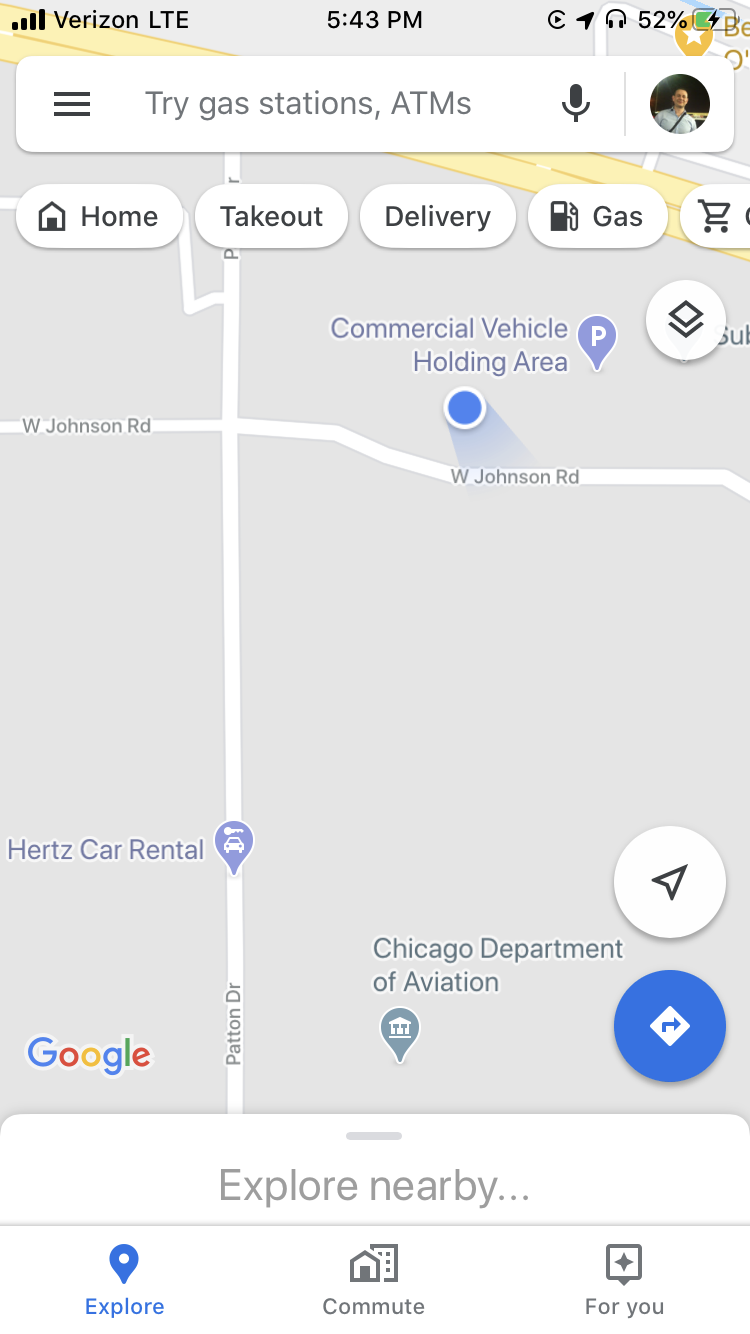The image is a detailed screenshot of a smartphone displaying a map application. At the very top, the phone's status bar shows "Verizon LTE" as the network provider, the current time, and several standard notification icons on the upper right. Below the status bar, there's a search bar featuring a burger menu icon on the left, a microphone icon on the right, and next to the microphone icon, a circular user profile picture. 

Directly beneath the search bar, a series of category buttons is displayed, each enclosed in white ovals. The categories listed include "Home," "Takeout," "Delivery," "Gas," and one additional, unspecified category.

The main body of the image is dominated by the map view itself. The map features white roads set against a backdrop of gray blocks representing different geographical areas. Locations are labeled in blue text and include points of interest such as "Commercial Vehicle Holding Area," "Hertz Car Rental," and "Chicago Department of Aviation."

On the map, a prominent white circle with an arrow pointing to the top right is visible, signaling a specific direction. Beneath this, a blue circle houses a diamond containing a right-turn arrow, indicating an upcoming turn.

At the bottom of the image, a tab labeled "Explore Nearby" is visible, offering options such as "Explore," "Commute," and "For You" directly below it, providing additional navigation and exploration functionalities.